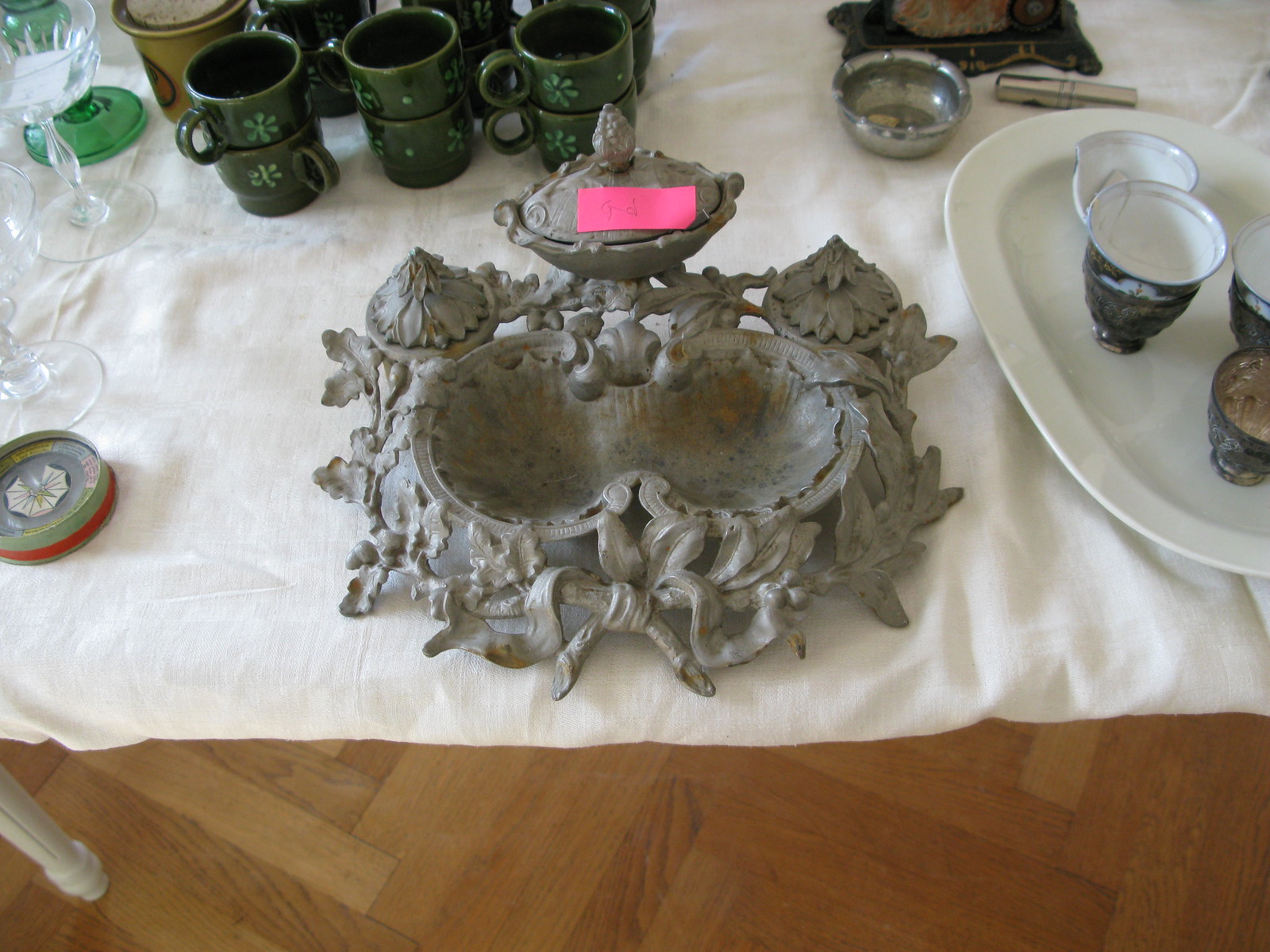A detailed gray-colored sculpture featuring an intricately designed double-bowl structure occupies the center of a white tablecloth-covered table with a wooden floor beneath. The sculpture's two small bowls display a rustic and blackened hue at their bases, separated by a minor hump and encircled by a ring. Surrounding this centerpiece are metal-shaped leaves. At the top of the sculpture is a removable gray pot lid, topped with a bulb-like handle, adorned with a pink sticky note inscribed with black lettering.

To the right of the main sculpture sits a white plate holding several cups that are black on the outside and white on the inside. Further in the background are objects suggestive of an antique or display setup, such as stacked dark green coffee mugs and wine glasses that appear to be crafted from clear glass or maybe plastic. Additionally, a small silver container, probably an ashtray, is visible. On the far left side of the table, a compass, adorned with green and red circles, can be seen amidst the arrangement of antique-like items.